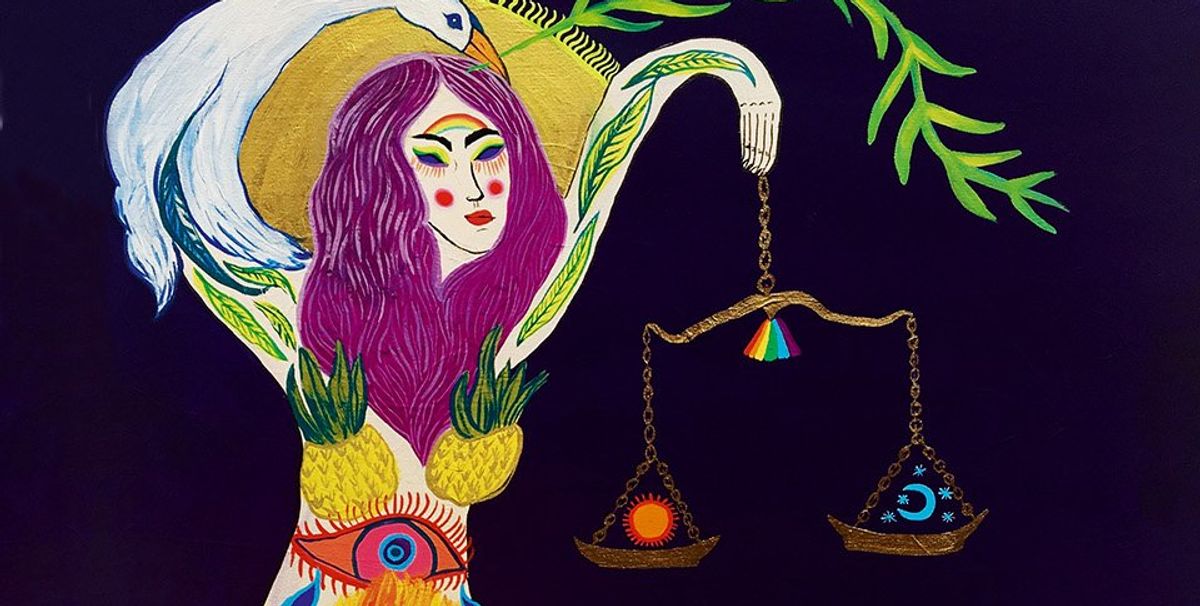The artwork features a striking depiction of a woman against a completely black background. Occupying the left side of the piece, the woman has long, flowing purple hair with white streaks, and a vibrant rainbow arching from one black eyebrow to the other. Her blue eyes are accentuated with red dots beneath them and a touch of yellow-green eyeshadow, while her lips are painted a deep red. The red circles on her cheeks add to the vivid color scheme of her face.

Her chest is modestly covered by two painted pineapples, their green-yellow leaves sprouting from the top. An intricately detailed eye adorns her stomach, surrounded by shades of orange, pink, and blue, complemented by red lashes and eyelid detailing. Below this, a flame-like design decorates her lower stomach, and she has yellowish marks and blue elements around her midsection.

Her right arm morphs into a white bird with an orange beak, carrying a leafy green branch tinged with yellow. Her left arm forms an arch, ending in a hand that holds a gold scale connected by chains. This scale features a sun, characterized by a yellow center and radiating red and orange lines, on the left plate, and a blue moon surrounded by stars on the right. Hovering above her is a sun-like object that casts a golden halo-like glow behind her head.

The combination of natural elements like leaves, fruit, and celestial bodies, along with the vivid and fantastical coloration, give the piece a surreal and captivating aura.